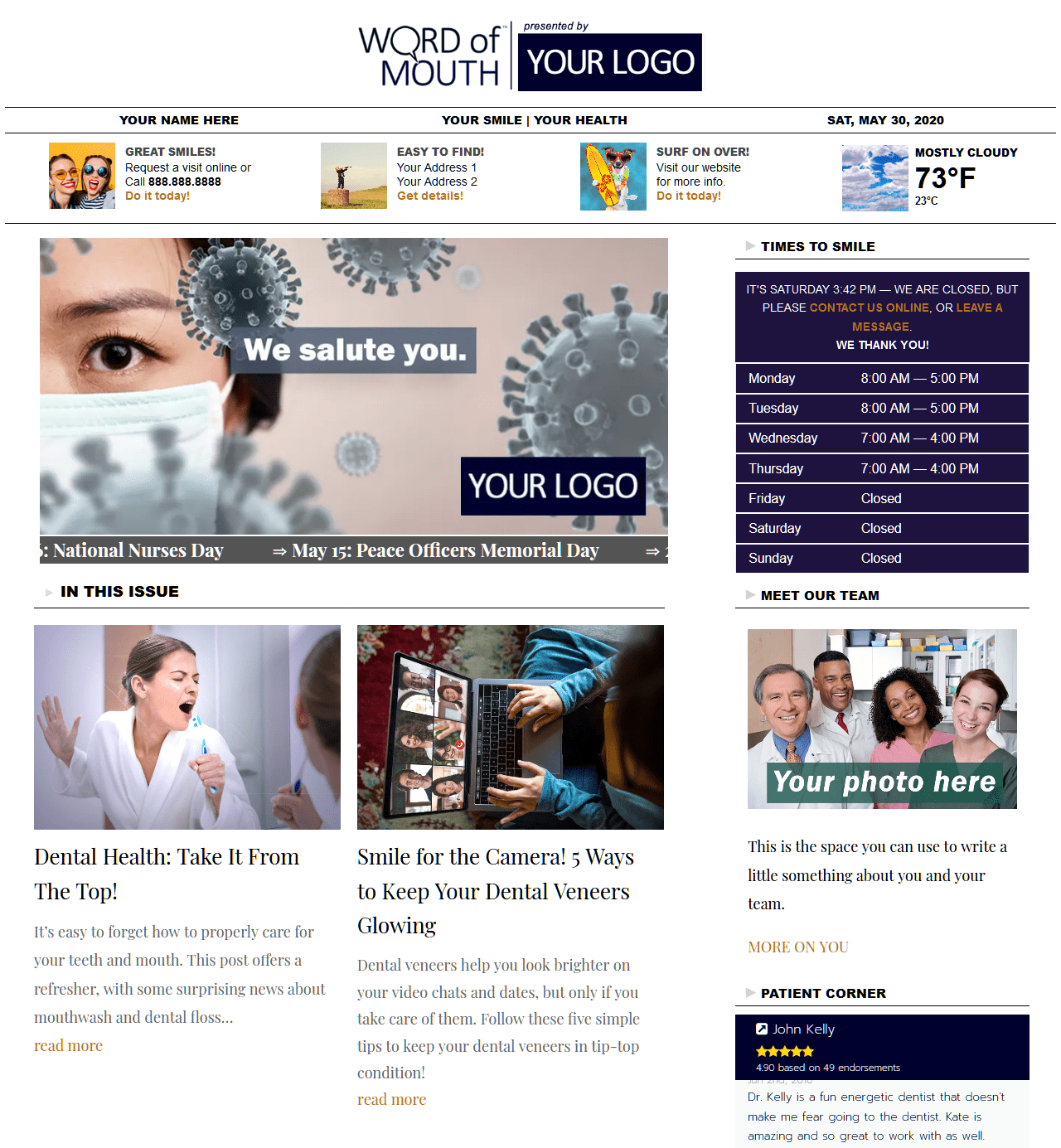This is a screenshot of a website featuring an all-white background. At the top center of the page, bold black capital letters spell out "ORAL HEALTH." Directly below this, in slightly smaller capital letters, reads "OF MOUTHS." A thin light black line separates these elements. Below this line, in smaller text, the words "presented by" are written.

A prominent black rectangle is placed beneath this text, with "YOUR LOGO" in bolded white capital letters inside it. Below this rectangle, there is a section with white space, framed by black at the top and bottom. In the left portion of this white space, "Your Name Here" is written. In the center, the phrase "Your Mile Your Smile and Your Health" appears, and on the right side, the event date "Saturday, May 30, 2020" is listed.

Moving down, the layout includes a row of four pictures. To their right, there is accompanying information and a phone number on one and a temperature on another. Below these images, there is a striking photo of the left side of a woman's face, highlighting her eye above a face mask, surrounded by grayish germs. The background of this section is tan. Across the middle of this image is the phrase "We Salute You" in white text.

In the bottom right corner, the "YOUR LOGO" appears again. To the right of the woman's photo, the phrase "Times to Smile" is displayed, followed by the days of the week indicating open hours: Monday, Tuesday, Wednesday, and Thursday.

On the left side of the page, beneath the photo, a section labeled "In This Issue" includes a brief description beneath two side-by-side images with associated headlines and paragraphs.

Finally, on the right side, below the open hours, a "Meet Our Team" section is displayed. It features a photograph of two women on the right and two men on the left, accompanied by a descriptive paragraph. In the bottom right corner, there is a blue rectangle with "John Kelly" inside it along with five stars, followed by another paragraph of information below.